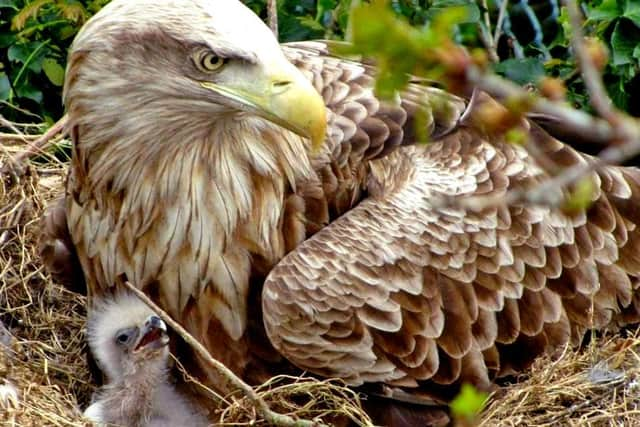This photograph captures a majestic adult eagle sitting in its nest, built from small twigs and a light brown grass-like material. The eagle, adorned with striking brown and white feathers, has its head turned to the right, highlighting its sharp, yellow-orange beak and one keen eye. Beneath the protective stance of the parent, an eaglet with grayish fluffy down and a tiny black eye gazes upward, its beak open in a plea. The nest is nestled within a dense area of greenery, with some blurred branches and buds appearing in the foreground, adding depth to the image. Hints of darker green foliage frame the background, giving context to the natural habitat.